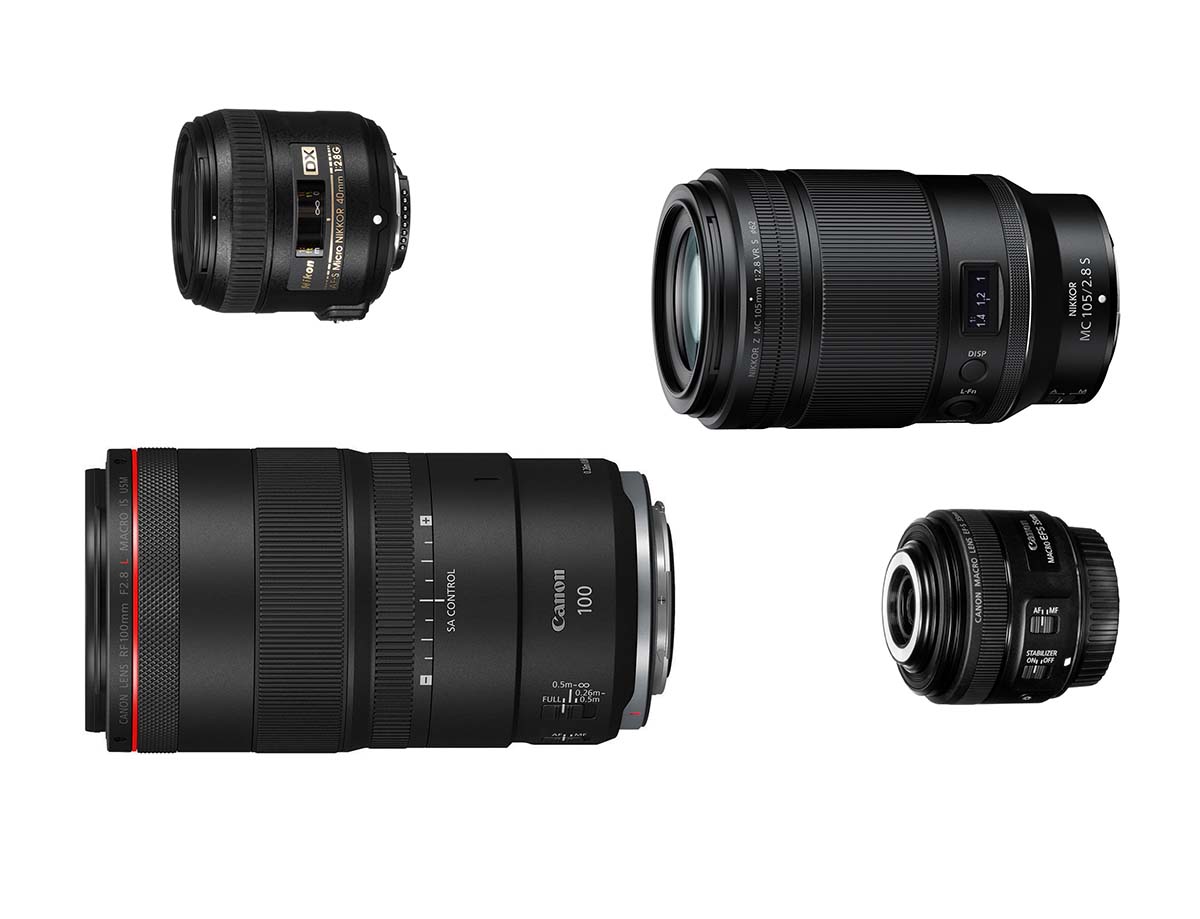This image features four distinct camera lenses arranged against a white background, showcasing their cylindrical shapes and black exteriors. The top-left lens is the smallest, labeled with "DX," though the rest of the writing is unclear. To its right lies a medium-sized lens, with indistinct text. On the bottom left, there is a large lens clearly marked for the Canon 100. Finally, the bottom right contains another small lens with illegible writing. The lenses, belonging to Canon and Nikon brands, bear additional details such as focal length and control information, hinting at their varied uses for different photographic needs.